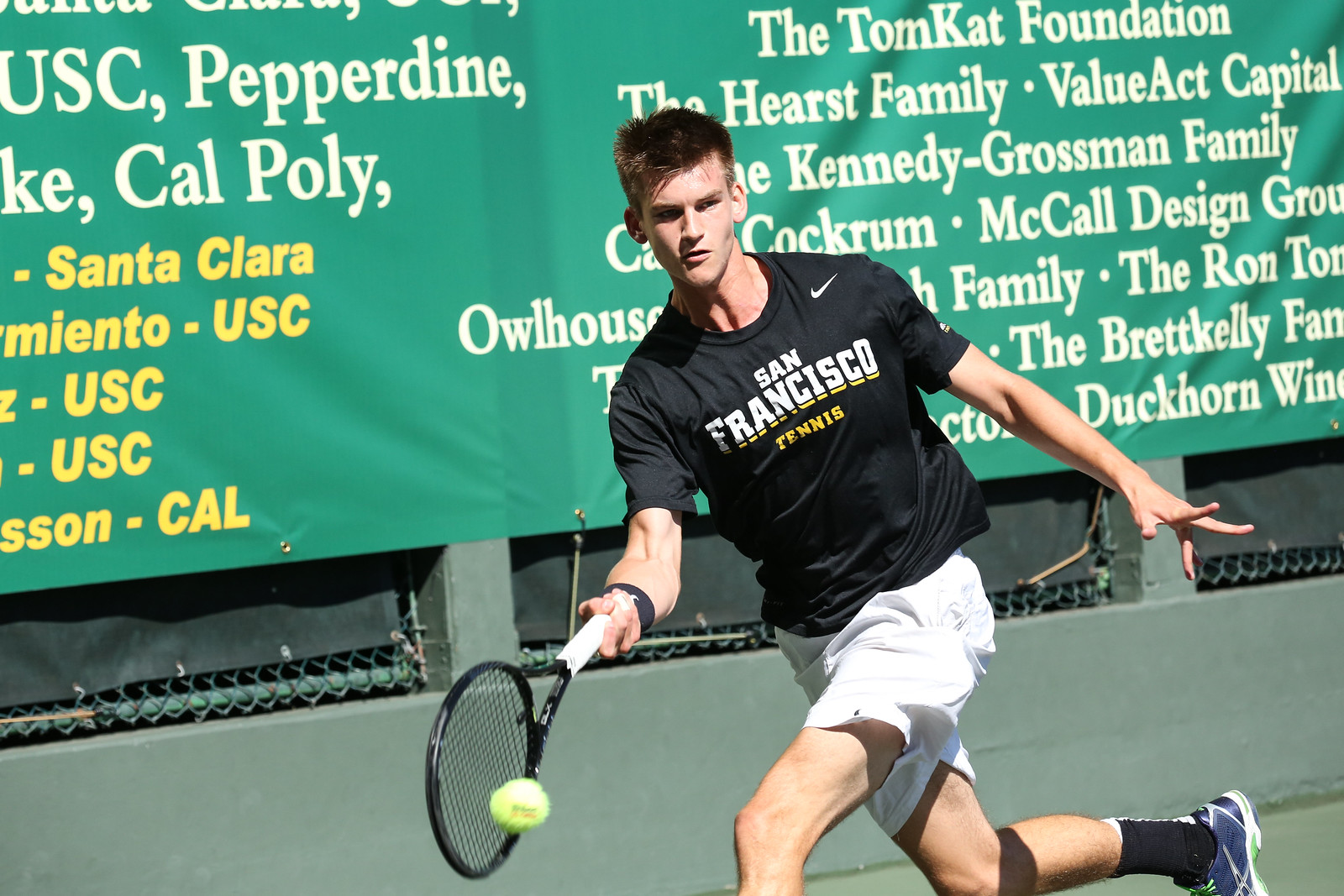The photograph depicts a young, light-skinned male athlete, likely a high school or college student, playing tennis on an outdoor court. He has short brown hair and an angular face, focused intently on the action. He is wearing a black Nike t-shirt with the words "San Francisco Tennis" emblazoned on it in white and yellow lettering, paired with white shorts and a black wristband on his right wrist. In his right hand, he holds a tennis racket poised to strike an incoming yellow tennis ball that is either about to hit or has just bounced off his racket. His body reflects dynamic movement: his left leg extends forward while his right leg bends back, and his left arm is outstretched with fingers splayed, perhaps in reaction to the ball’s trajectory. He dons black socks and purple Nike running shoes.

The backdrop includes a protective netting and a chain-link fence. Prominent green banners feature white and yellow text, listing multiple California college names such as USC, Pepperdine, Cal Poly, and Santa Clara. Additionally, there are numerous sponsor names in white lettering against the green background, some partially obscured by his figure. These include notable names like the Hearst Family, Value Act Capital, the Tomcat Foundation, and the Brett Kelly Family, among others. The image captures a moment in what appears to be a tennis tournament, evident from the competitive stance of the player and the numerous sponsor names supporting the event.